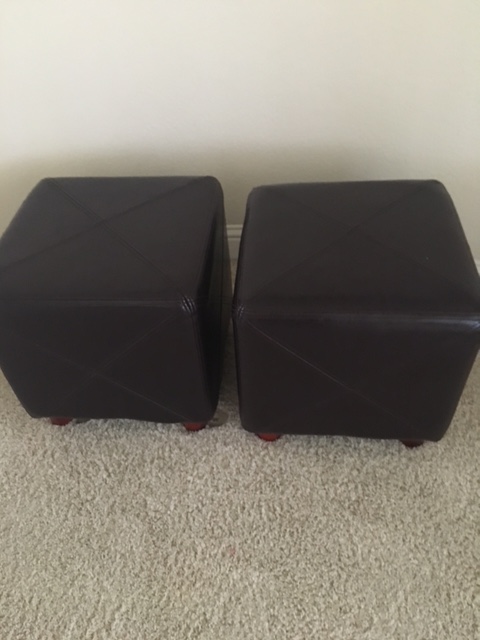The image showcases a poorly taken, low-resolution, color photo captured from a standing perspective, looking down toward the space between a wall and a carpeted floor. The floor features medium-length, white carpeting. Dominating the center of the image are two square, black leather or faux leather ottomans placed side-by-side. The ottomans, mistaken by some for end tables, sport fine-lined X-shaped stitches on both the tops and sides. Each ottoman stands on small, dark brown legs that resemble stumps. The background includes a light gray wall with a white baseboard visible above the carpet, serving as a simple backdrop to the featured furniture pieces. The photo cuts off the far corners of the ottomans, emphasizing their presence within the context of the room.